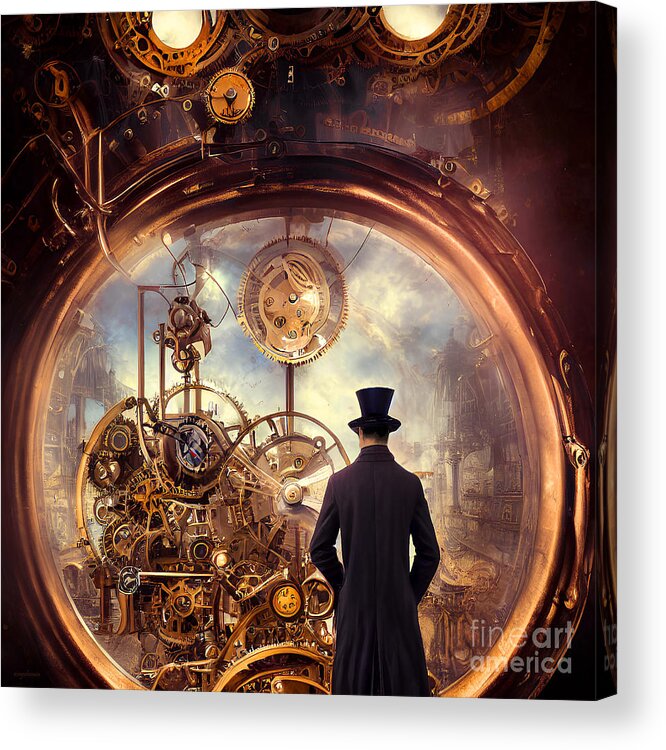The image appears to be a steampunk-inspired painting or AI-generated artwork featuring a large, circular window set in a predominantly dark, rustic, and purple-brown backdrop. Surrounding the window and continuing within it are numerous golden gears and mechanical devices, though the details of the gears appear somewhat erratic and underdefined, likely added for artistic effect. The focal point of the image is the back silhouette of a man clad in a long, dark coat and a black top hat, standing before the window and gazing out at the complex network of interconnected, gold-colored cogs and tube piping that extend into a blue sky with scattered clouds. The scene conveys a blend of intricate machinery and evocative steampunk aesthetics. In the bottom right-hand corner, the image is marked with a faded, transparent watermark reading "Fine Art America."